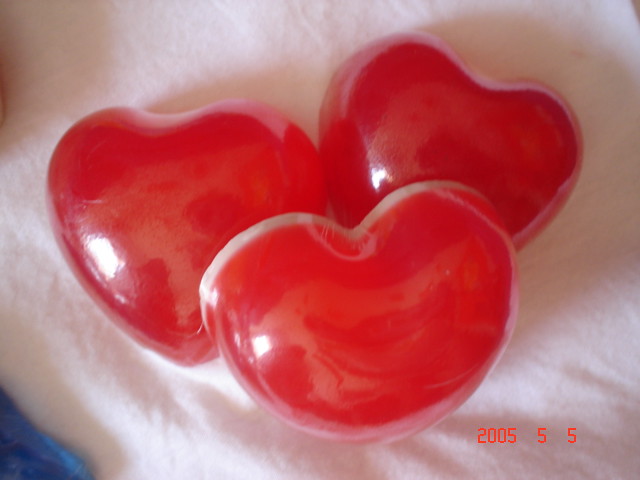This is a detailed photograph showcasing three bright red, shiny hearts, possibly made of glass or plastic, giving them a candy-like appearance. The hearts are highly reflective, capturing light and possibly reflecting the camera used to take the picture. They are arranged with two hearts nestled side by side at the bottom, while a third heart is positioned on top, slightly lower, creating a layered effect. The hearts are displayed on a smooth, white cloth background, reminiscent of a T-shirt or napkin with no visible pattern. In the bottom left corner, a small triangular piece of blue cloth is visible. Additionally, the bottom right corner features a red-font timestamp that reads "2005 5 5."